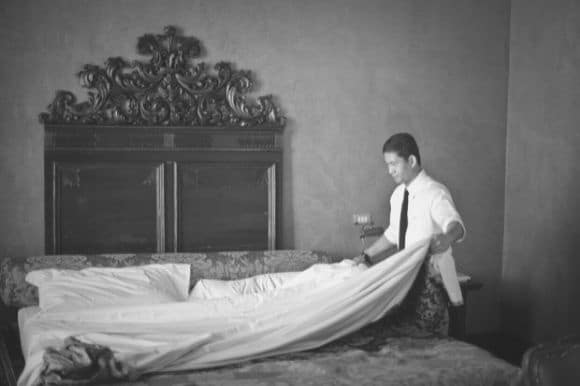This black-and-white, horizontal rectangular photograph captures a man meticulously making an ornate bed, possibly in a luxurious hotel room or a grand home. The backdrop features a highly detailed headboard with an intricate spiral scroll design. The man, who seems to have a darker complexion that suggests he could be of Asian or Latino descent, has short black or dark brown hair. He is attired in a white dress shirt with the sleeves rolled up to his elbows, a black tie, and decorative pants, with the tail of his shirt hanging out. He appears to be holding and adjusting a white sheet on the double bed, which also has two white pillows and a brocade-patterned bed covering. The bed's headboard stands out with its unique design, and there's mention of a cabinet with closed doors behind it, though the walls themselves are bare. The image quality is somewhat low resolution, but the man's careful attention to making the bed and the room's ornate features remain clear.